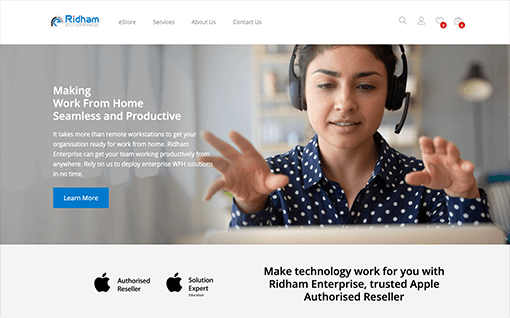**Detailed Image Caption:**

This image is a screenshot of a web page. At the top left corner, the word "RIDHAM" is prominently displayed in blue letters. Directly beneath "RIDHAM," there is a gray, blurred word that is unreadable. 

The navigation menu spans from the left to the right across the top of the page. The menu items are:
1. "E-STORE" in gray letters to the right of "RIDHAM."
2. "SERVICES" to the right of "E-STORE."
3. "ABOUT US" to the right of "SERVICES."
4. "CONTACT US" to the right of "ABOUT US."

On the far right-hand side of the page, the top row includes various icons:
1. A magnifying glass icon representing the search function.
2. An outline icon of a person symbolizing the user profile.
3. A heart icon with a red notification circle in front of it.
4. A suitcase icon, also with a red notification circle.

Beneath this header, there is a prominent image of a lady. She appears to have disproportionately short arms and is wearing a blue shirt with white polka dots. The woman is donning headphones and has brown hair, suggesting she may be white or Hispanic.

To the left of her image, in bold white letters, a motivational message reads:
"MAKING WORK FROM HOME SEAMLESS AND PRODUCTIVE. IT TAKES MORE THAN A REMOTE WORKSTATION TO GET YOUR ORGANIZATION READY FOR WORK FROM HOME. RIDHAM ENTERPRISE CAN GET YOUR TEAM WORKING PRODUCTIVELY FROM ANYWHERE. RELY ON US TO DEPLOY WORK FROM HOME SOLUTIONS IN NO TIME."

Below the text, there is a blue button labeled "Learn More."